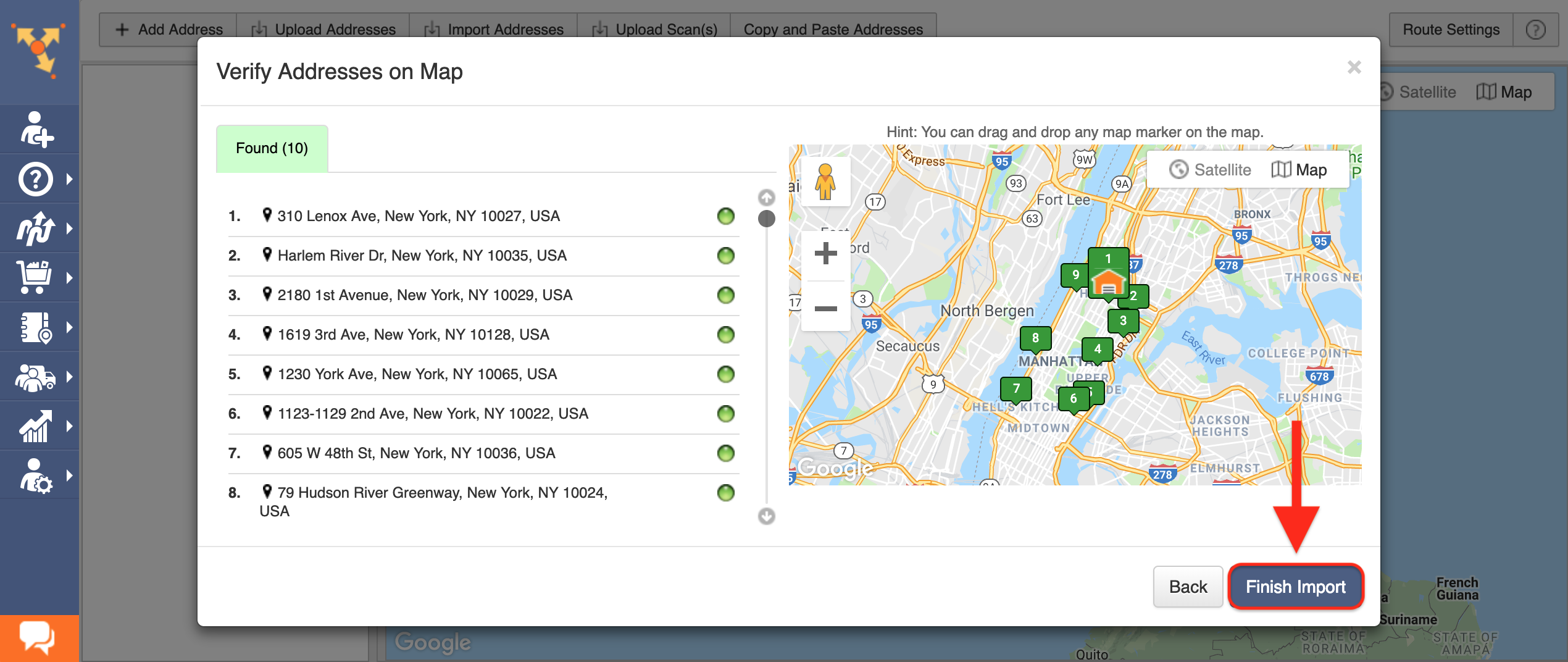This map image displays several verified addresses across a detailed city layout. Key locations highlighted include North Bergen, Circuses, Manhattan, College Point, Flushing, Jackson Heights, Elmhurst, Hell's Kitchen, and Midtown. The map features interactive elements that allow users to drag and drop markers to different spots. Prominent colors on the map are green, white, and red, creating a vivid visual contrast. Additionally, a red arrow points towards a specific area, adding emphasis for navigational ease.